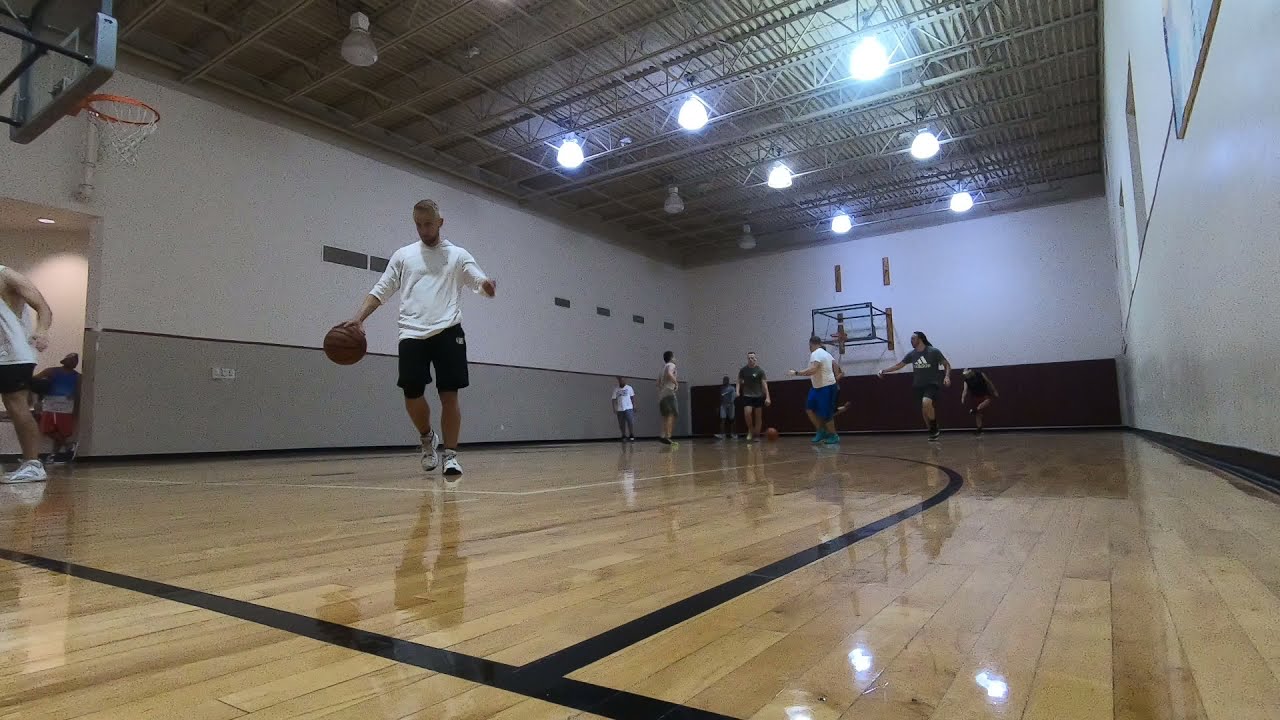The image captures a dynamic scene inside a gymnasium where a casual basketball game is unfolding. The shiny hardwood court displays its black markings, delineating the three-point line and out-of-bounds areas. Centered on the action, a middle-aged man in a long sleeve white shirt and black shorts is dribbling the ball towards the hoop. Close to him, on the left side of the frame, another man in a white short sleeve shirt is partially off-screen near a water fountain. In the background, a diverse group—comprising men, women, and a little boy in a white shirt—are either running or appear to be gathering around a basketball at the free throw line. The gym's white walls juxtapose with the high ceiling's hanging lights, emphasizing the narrow, elongated nature of the space. Overall, the image portrays a fun, non-competitive environment with around six people scattered across the court, likely engaged in a friendly three-on-three pickup game.